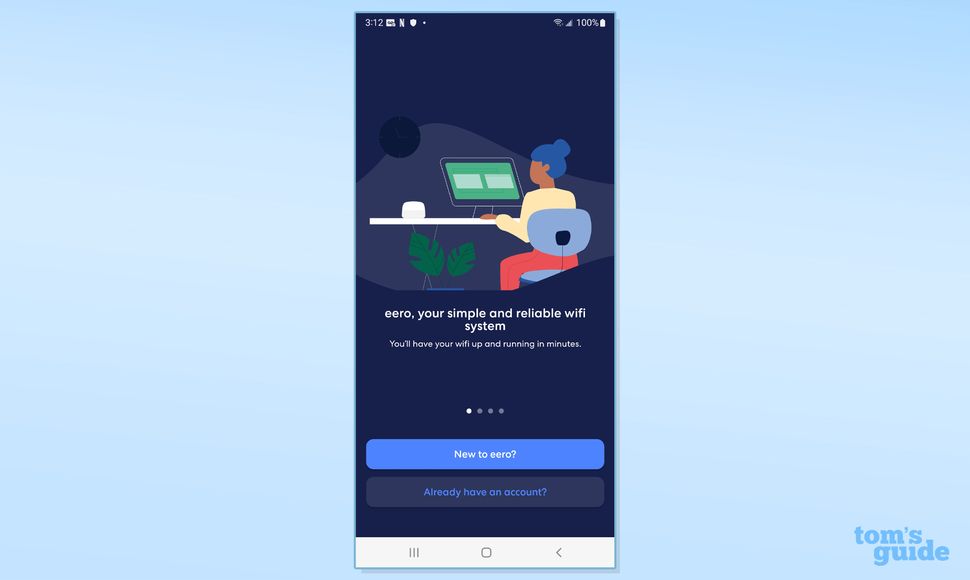The image features a light blue background. In the center is a smartphone displaying a screen with a dark blue background, indicating the time as 3:12 and a battery level of 100%. On the screen, there is a promotional image showing a woman seated in a blue chair at a white desk, working on a computer. The screen text reads, "Eero: Your simple and reliable Wi-Fi systems. You'll have your Wi-Fi up and running in minutes."

Below this message, there are four navigation dots, with the first one highlighted in white. Beneath the dots, a blue box offers options with text that reads, "New to Eero" and "Already have an account." The bottom section of the screen is dark blue, featuring white text elements, including an icon with three horizontal lines, a box, and a left arrow.

Additionally, "Tom's Guide" is written in white in the bottom right corner of the light blue background. The overall impression is that Eero provides an easy setup for Wi-Fi, emphasized by the imagery and streamlined interface to get users connected within minutes.